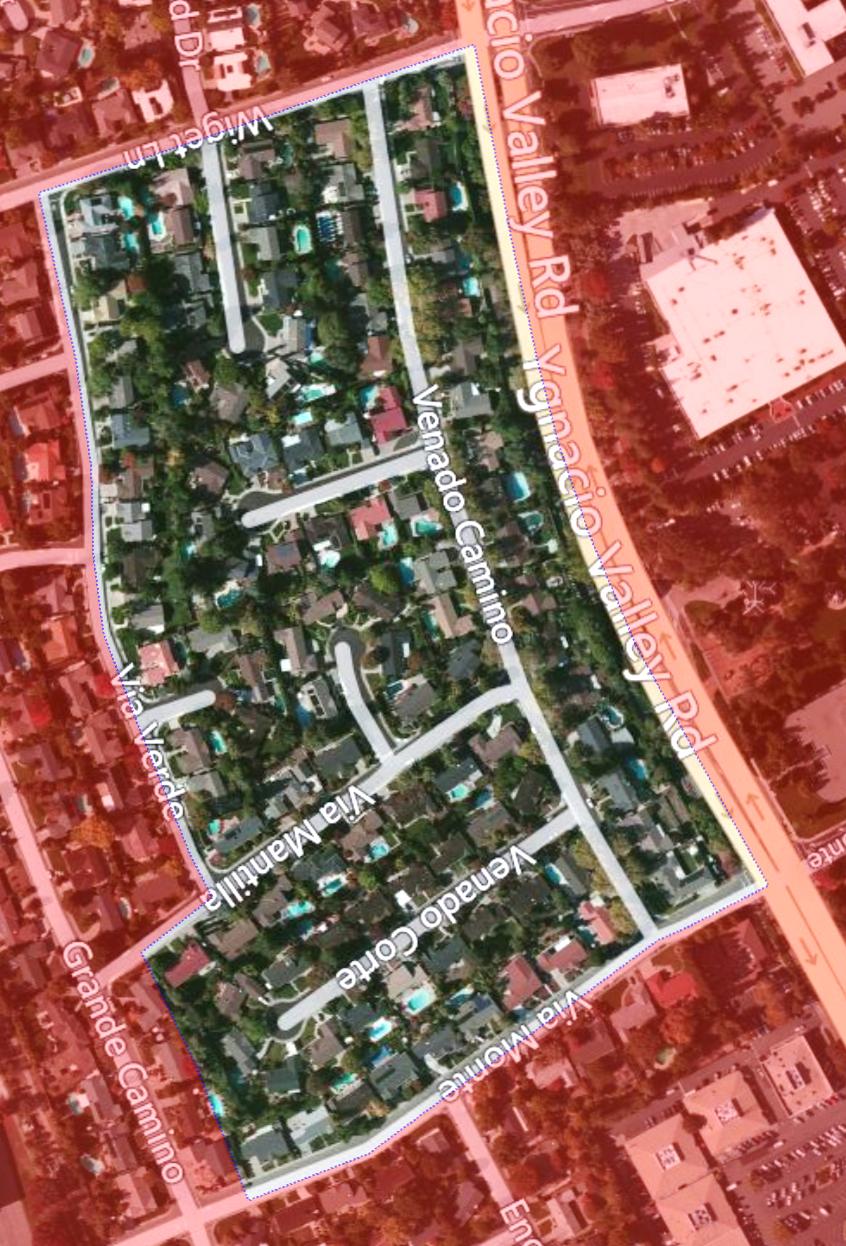This image is a detailed satellite view of a neighborhood captured from Google Maps. The central focus is highlighted by a clear red outline encompassing the vibrant, full-color area. Surrounding this neighborhood are various streets and notable landmarks, including the major thoroughfare, Bonacito Valley Road. Inside the red-outlined neighborhood, the primary roads include Venado Camino, Villa Mantilla, Villa Verde, Villa Monte, and Wiget Lane.

The neighborhood is characterized by a mix of residential houses, many of which feature pools. The green landscape is dotted with numerous trees and well-maintained lawns, contributing to the area's lush appearance. The high-resolution satellite view also showcases the layout of the buildings and the overall urban planning of the vicinity, highlighted by the presence of gray, yellow, and straight map lines that demarcate various streets and properties.